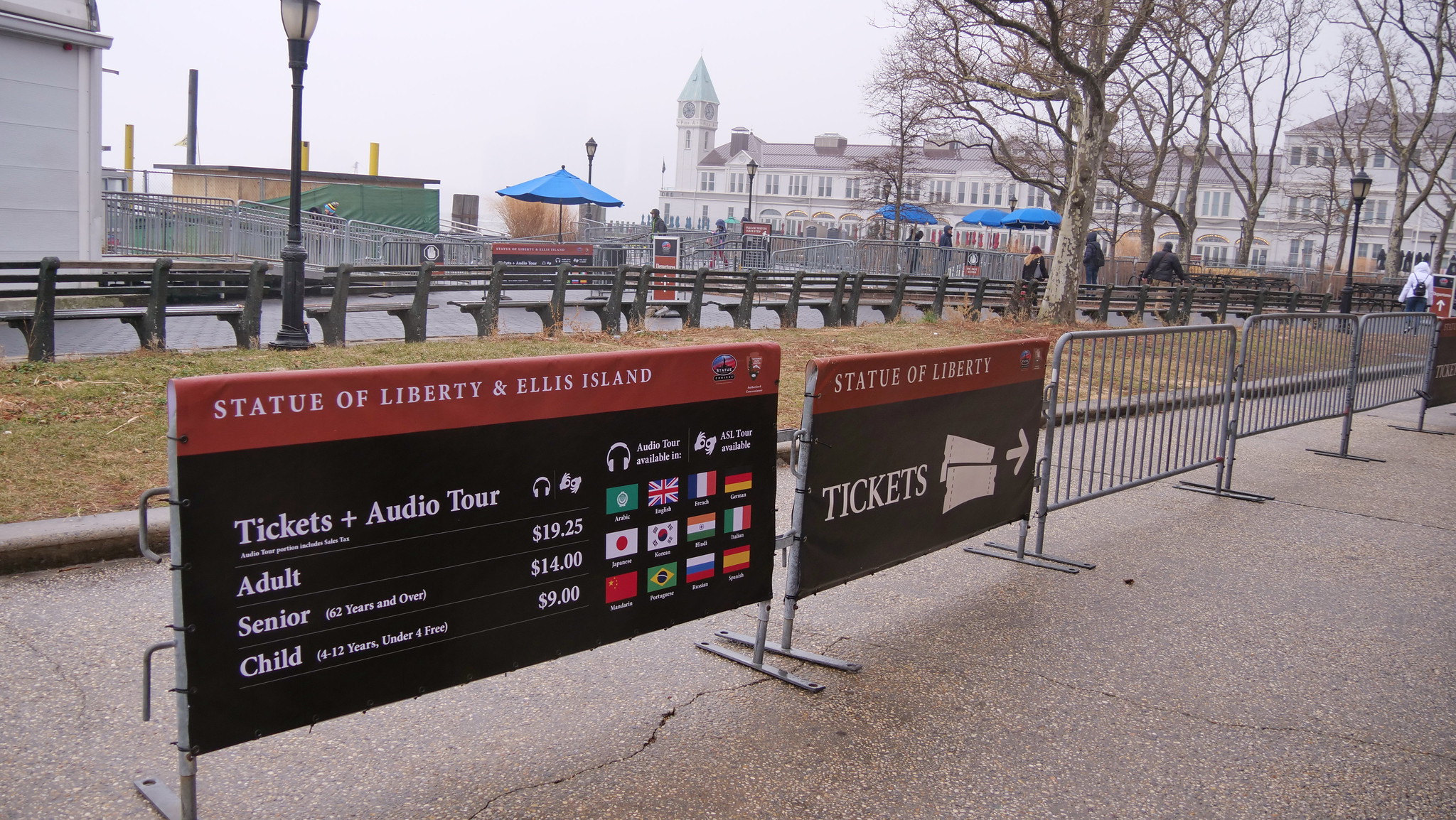A bustling walkway leading to the iconic Statue of Liberty and Ellis Island is depicted. Right in the foreground, metal gates guide the visitors towards a prominent, black advertisement board. The board features stark white lettering that reads "Statue of Liberty Ellis Island" on a striking red strip at the top. Below this, details about ticket prices for adults, seniors, and children, along with options for an audio tour, are clearly outlined in white text. 

Adjacent to this sign, another similar display appears, repeating the "Statue of Liberty" text on a red strip, with “TICKETS” boldly written in white capital letters against a darker background. This sign also includes two small images of ticket stubs and an arrow pointing to the right, directing visitors further along the path.

This area is segmented with three additional metal guardrails, all situated on a stone-like pathway. To the side of the walkway, a grassy expanse can be seen, dotted with an orderly row of wooden benches, all aligned in a neat sequence. Beside the benches, there is a body of water or possibly a dark road, though it is difficult to ascertain its exact nature from the image.

In the distance, barren trees stand tall, framing a backdrop of white buildings that stretch into the horizon, with a steeple peeking out on the left side, completing this scenic view of the bustling pathway leading up to one of America’s most treasured landmarks.